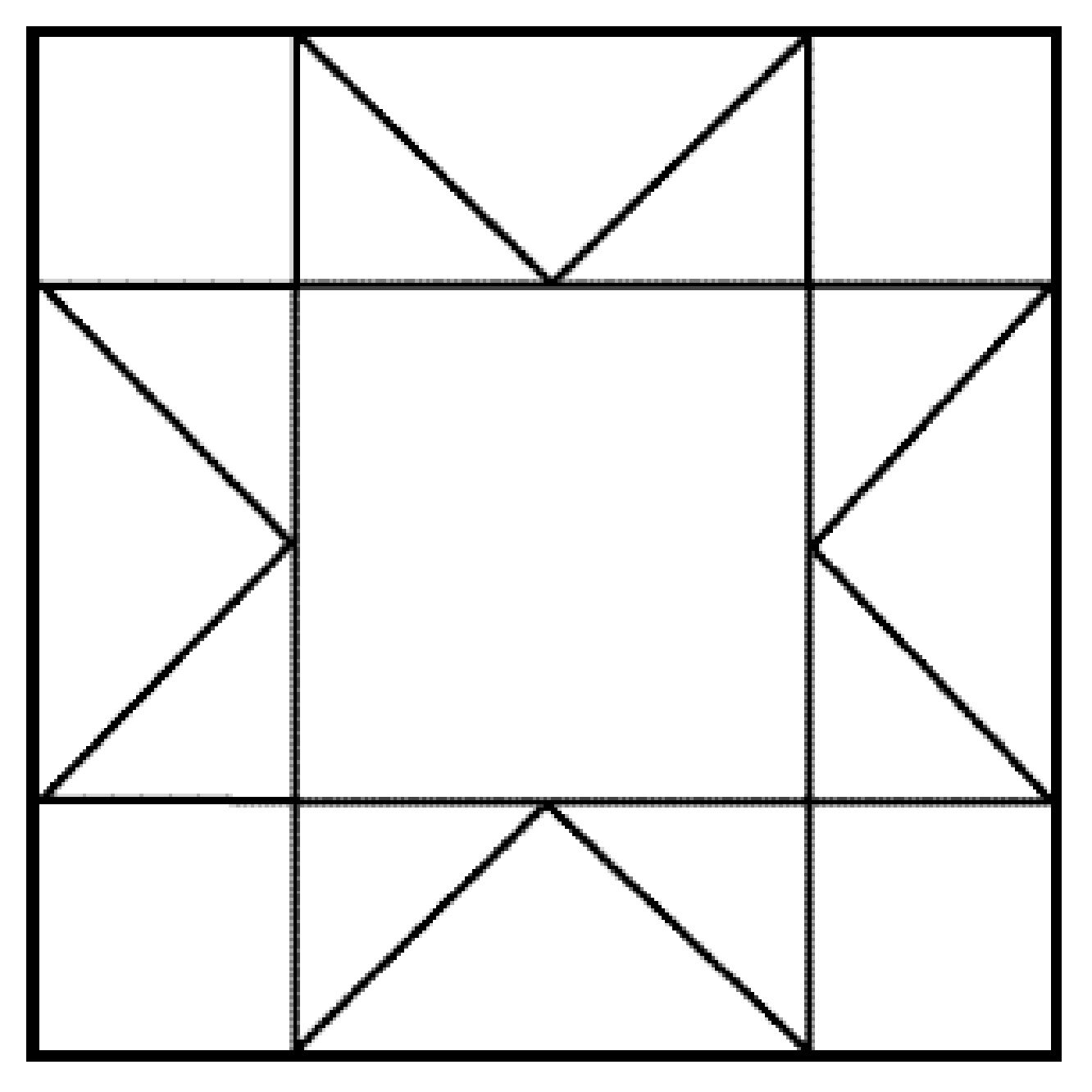This vector image features an intricate geometric pattern set against a pristine white background. At the heart of the design is a large central square, which encases a smaller square perfectly positioned at its center. Each corner of the central square is marked by four very small squares, strategically situated at the top left, top right, bottom left, and bottom right corners.

Connecting the small squares, rectangular areas stretch across the sides of the large square. Each rectangle is ingeniously segmented by a prominent V shape, effectively dividing it into three distinct triangles. This V-shaped division is mirrored in all four rectangular areas, creating a harmonious and symmetric geometric pattern that captivates with its precision and simplicity. The entire composition resonates with balance and meticulous design, making it a striking visual presentation.